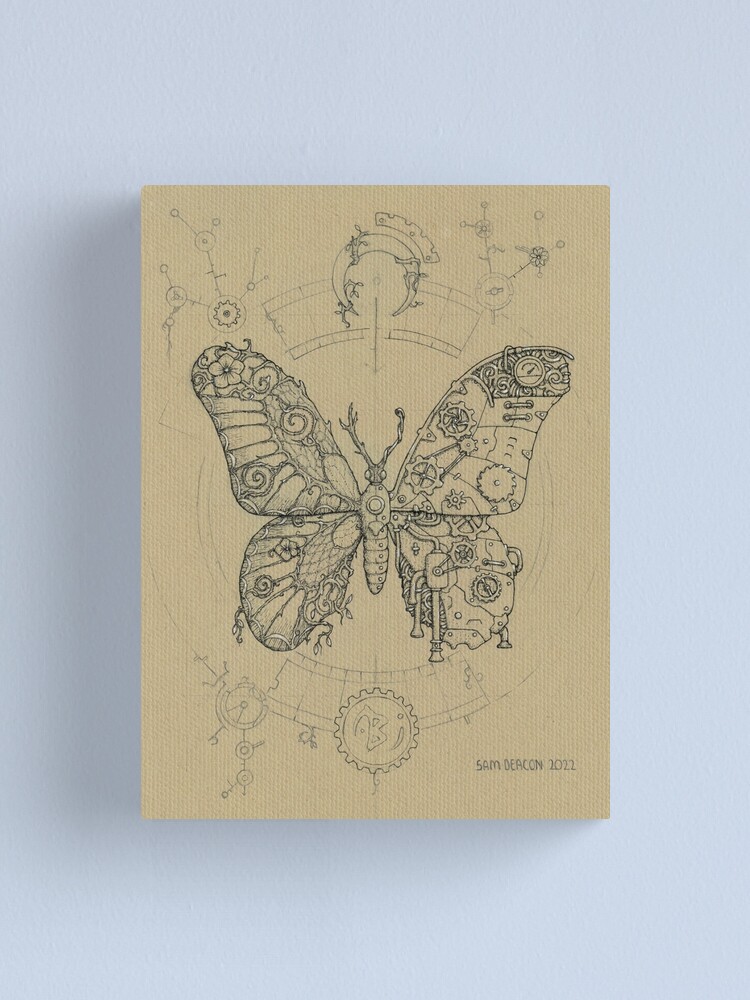This intricate pencil-sketch by Sam Deacon from 2022 features a mesmerizing depiction of a butterfly, drawn on a white canvas with a cardboard-like texture. The butterfly's wings are a stark contrast between the organic and the mechanical: the left wing is adorned with flowers, vines, and other natural elements, while the right wing is an assemblage of gears, cogs, pipes, and sheet metal with rivets, symbolizing machinery. The body of the butterfly is a fusion of these two worlds, incorporating both natural swirls and mechanical shapes like nets and clocks. The antennae reflect this dichotomy too, resembling branches on one side and twisted wires on the other. Surrounding the butterfly are various detailed elements including a large gear with the letter 'B' below it, a crescent moon entwined with vines above, and compasses flanking the sides. Additional mechanical and drafting elements, such as small circles, curved rulers, and gears, add to the complexity, creating a captivating blend of technology and nature. Sam Deacon's signature and the year '2022' are inscribed in the bottom right corner.